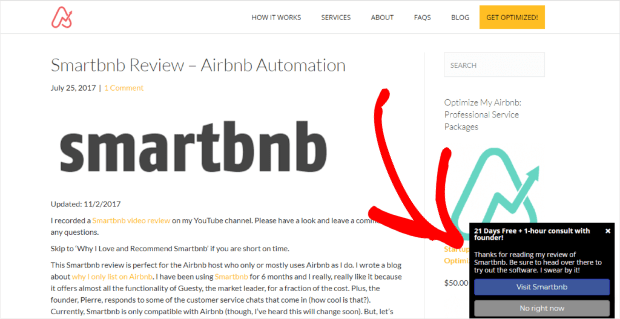Top left of the image displays the AirBnB logo accompanied by the heading "How it works." Below this are menu options: Services, About, Facts, Blog, and Get Optimized, each highlighted in yellow rectangles. 

A section titled "SMARTBNB Review - AirBnB Automation" is dated July 25, 2016, and features one comment under the name SMARTBNB. It continues with an update, "Update 11," and a date, "Select Tuesday, 2017." 

The narrative below elaborates: “I have recorded a SMARTBNB video for my YouTube channel. Please take a look and get to know why I love and recommend SMARTBNB, especially if you’re short on time. This SMARTBNB review is perfect for the AirBnB community focused on optimizing their listings. 

Having used SMARTBNB for 6 months, I can attest to its comprehensive features and cost-efficiency. The founder appears very responsive, often engaging in numerous chats—how cool is that? Currently, SMARTBNB closely resembles AirBnB, though I’ve started using bullet points to organize information better. 

A highlighted red arrow points towards an offer: '21 days free plus 1-hour consultation with a friend.’ 

Thanks for reading my review of SMARTBNB. Be sure to thoroughly review and try out the software I endorse. Visit SMARTBNB. Note the white background in the image.”

![Image: AirBnB logo and SMARTBNB review details, including text, highlights, menu, review dates, and special offer](link-to-image).